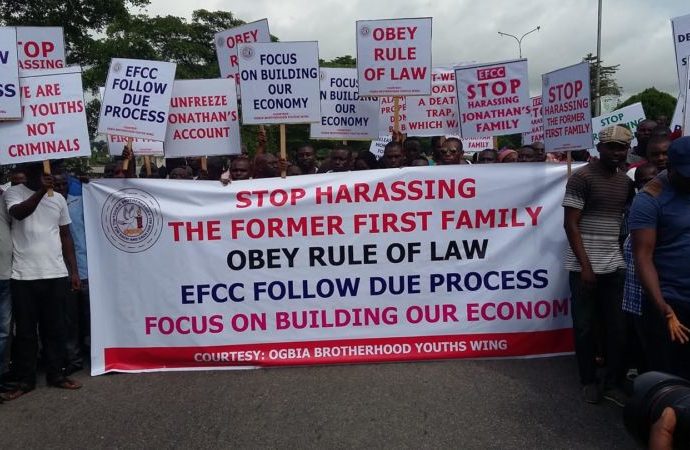The photograph captures a lively protest rally on an overcast day, with grayish-white clouds casting a muted light over the scene. A diverse group of predominantly brown-skinned men, many sporting very short hair, stand prominently. In the foreground, they hold a substantial white canvas banner, approximately 5 feet high and 15 feet wide, emblazoned with a mix of red, black, blue, and dark pink letters. The banner reads: "Stop harassing the former first family, obey rule of law, EFCC follow due process, focus on building our economy. Courtesy: Ogbia Brotherhood Youth Swing." Behind the banner, several protesters hold up white square signs on sticks, containing messages in either red or blue letters that echo the banner's call for justice and due process. The background features some trees and metal light poles. Additionally, in the lower right corner, one can spot a person with a camera lens, capturing the fervor of the event. This contemporary photograph vividly illustrates the determined spirit of the participants advocating for their cause.